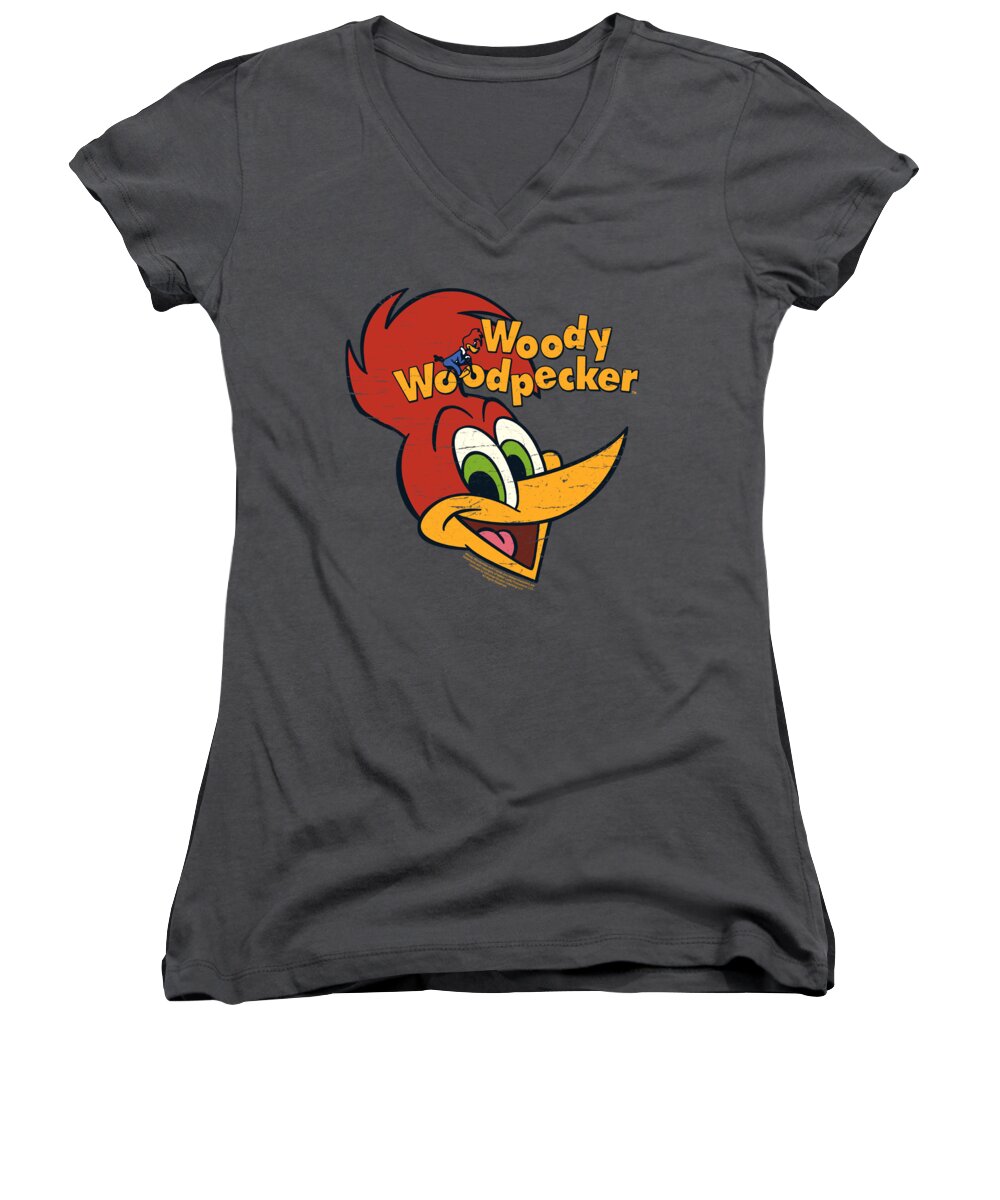This top-down photograph showcases a women's short sleeve, v-neck t-shirt, neatly laid on a flat white background. The t-shirt is a dark, rich gray with a subtle bluish tint. At the center of the shirt, there is a vibrant cartoon illustration of Woody Woodpecker. Woody Woodpecker's head, featuring his characteristic green eyes, red hair, and orange beak, is smiling broadly with his mouth open, revealing his tongue. Above Woody's head, the text "Woody Woodpecker" is displayed in unevenly spaced letters that mimic an undulating plane. Notably, in the word "Woodpecker," the double O's are transformed into bicycle wheels with a bike frame, and Woody Woodpecker is depicted pedaling atop this makeshift bike, humorously riding on his own name. The top of the t-shirt is narrower, flaring slightly at the bottom, suggesting a design for women. The overall presentation of the t-shirt, with its detailed graphic and playful design elements, hints at a photo intended for a clothing website or magazine.